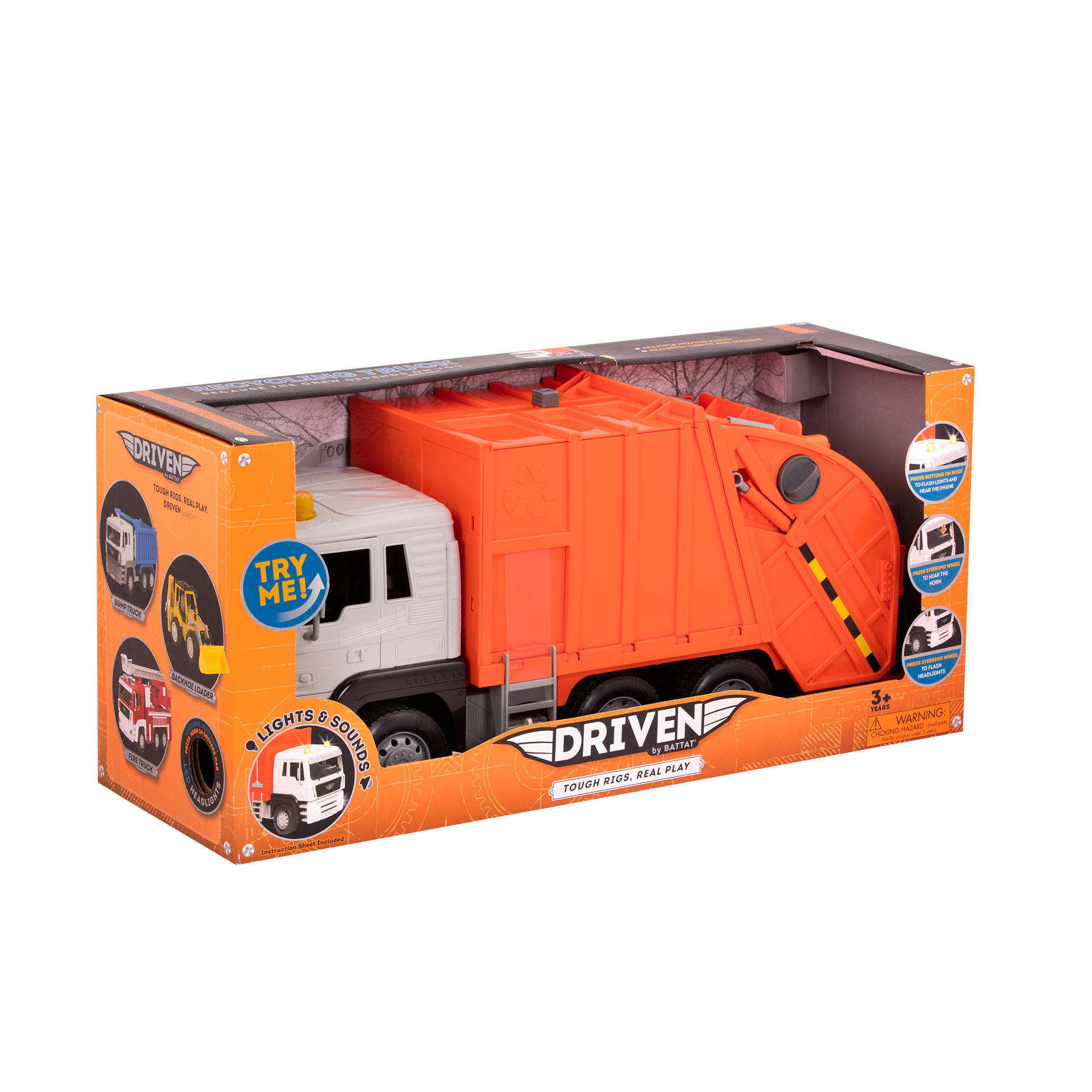The photograph depicts a large child's toy packaged in its original box, appearing typical of what might be found in stores like Target. The toy is a robust truck, designed to resemble a garbage truck, with a distinctive orange container at the back. This container features a curved section and a hydraulic mechanism for opening the lid. The truck's cabin contrasts in a white color. The box itself has an orange exterior and a grayish interior, prominently displaying the brand "Driven" along with its tagline "Tough Rigs, Real Play." The packaging also indicates the toy is suitable for ages three and up and showcases additional truck designs available in the same series, including a tractor with a plow and a fire truck, depicted in circular icons on the bottom left side of the box.